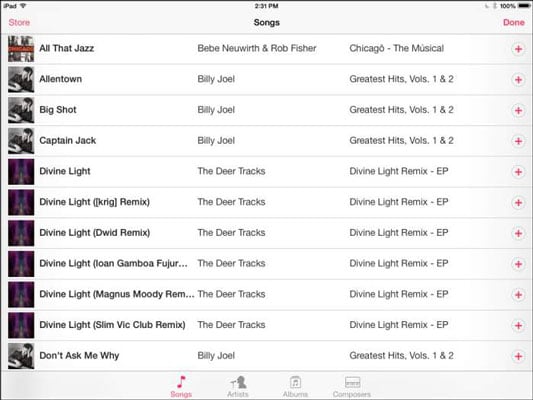Screenshot of an iPad taken at 2:31 PM, showing 100% battery, presenting a playlist with the title "Store Songs" in red, labeled "done." The playlist includes:

- "All That Jazz" by Bebe Neuwirth and Rob Fisher from "Chicago the Musical"
- "Allentown" by Billy Joel from "Greatest Hits Volumes 1 and 2"
- "Big Shot" by Billy Joel from "Greatest Hits Volumes 1 and 2"
- "Captain Jack" by Billy Joel from "Greatest Hits Volumes 1 and 2"
- "Divine Light" by The Deer Tracks from the "Divine Light Remix EP" (listed as "Divine Light (King Remix)")

Each song title has a plus sign next to it, highlighted in red.